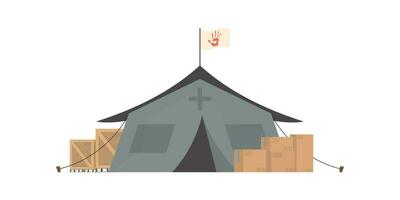This is a small, stylized illustration of a large, gray-green military-style tent. The tent features a cross above its entrance flap, which is open to reveal a dark interior. There are simplistic mesh windows indicated on either side. At the top of the tent, there is a white flag adorned with a red handprint, which appears almost cartoonish, as though someone had stamped their painted hand onto the fabric. Surrounding the tent are several crates, some stacked, suggesting supply storage. The tent is pitched with guy lines, though they appear slack. The entire image is rendered in a monochromatic, icon-like style against a white background, giving it a simplistic and somewhat minimalist appearance.